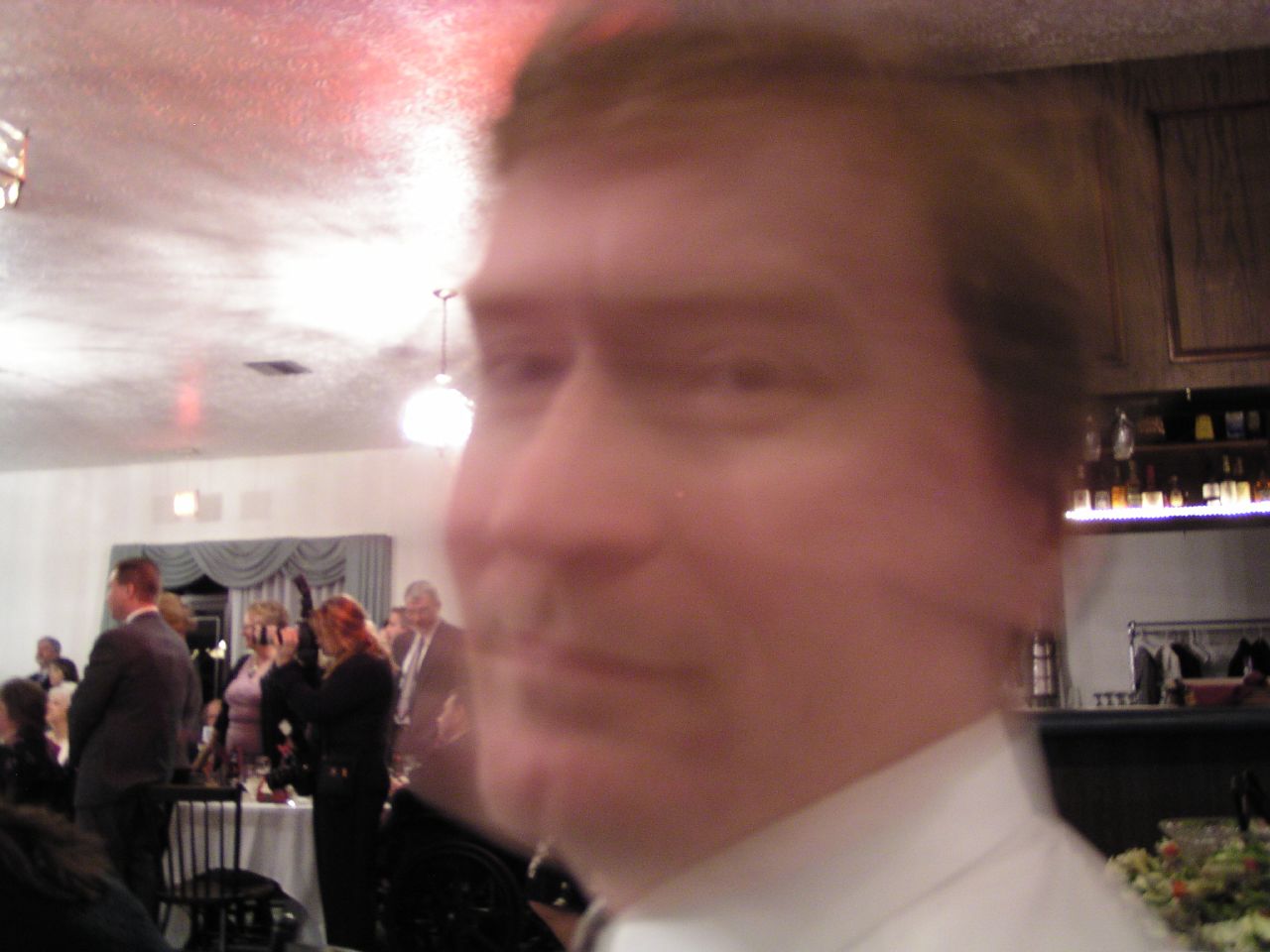This image captures a bustling indoor celebration, perhaps a dinner party or a gathering, set in a room with a blend of homey and formal elements. The foreground is dominated by a very blurry male figure dressed in a white shirt and a black tie, with distinguishable orange hair, who appears to have moved just as the picture was taken. The background, however, is much clearer and is filled with details:

To the left of the man, there is a setting that looks like a kitchen area with dark cabinets, possibly a dark-colored countertop, and various items like spices, drinks, plates, and bottles. The far background reveals a cozy, yet elegant space featuring tables dressed with white tablecloths and black chairs. These tables are adorned with some items and possibly food, though the specifics are not clear.

Surrounding the tables are numerous people, both male and female, dressed in a range of outfits including black, pink, and gray. Some are standing, others are sitting, all seemingly engaged in the celebration. Behind them, a wall bearing gray multi-layered drapes crosses through a doorway, enhancing the room's elegant atmosphere. Adding to the festive ambiance is a chandelier hanging from the ceiling, whose light radiates blurrily across the scene, creating an inviting glow.

Overall, the image portrays a lively and inviting gathering with a mix of detailed surroundings and a dynamic, albeit blurry, foreground figure.